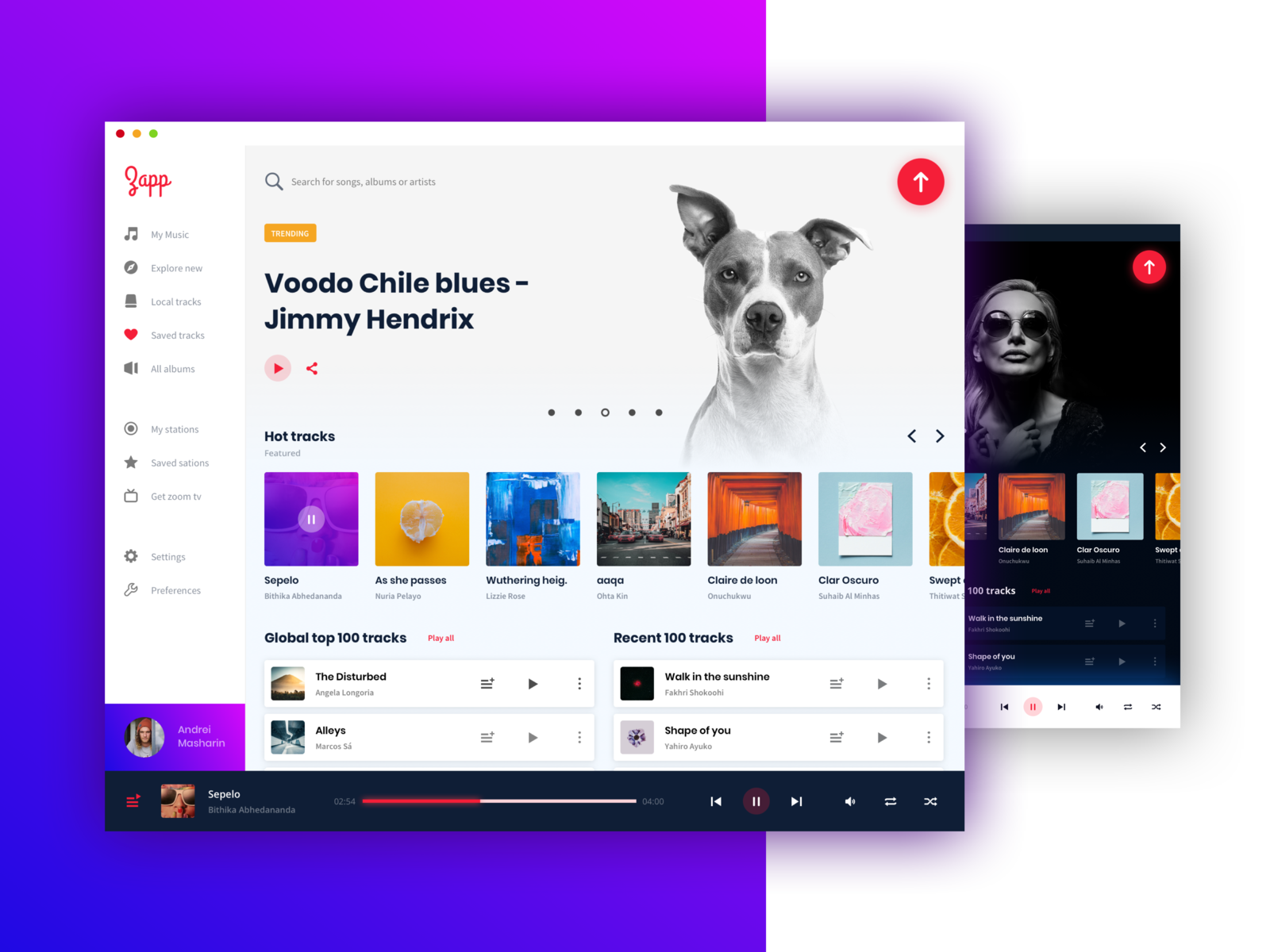The image showcases a vibrant, multifaceted website interface for a platform called "Zapp." The main website screen is overlaid on a colorful, gradient background that transitions from bright blue to bright purple in the upper-right corner, casting a vivid hue across the page. On the left side of the background, a rectangular section adds to the layered design.

To the right of the main screen, partially visible, is another overlay with a black background. This section features a black-and-white photo of a woman wearing sunglasses, possibly a musical artist, surrounded by various thumbnails of album covers, and controls including play, pause, and settings icons.

The focal point of the main interface is the Zapp website title, presented in a striking red script that evokes the style of Zatarain's food products. This primary webpage has a clean white background, dominated by a prominent black-and-white photo of a mixed-breed dog (possibly a pitbull or boxer mix) with one ear down and the other up. Adjacent to the dog’s image are the words "Voodoo Child Blues by Jimi Hendrix," accompanied by a red circle featuring an upward-pointing white arrow, likely indicating an option to upload the song.

Below this section, the website highlights a "Hot Tracks" area featuring a row of thumbnail images of various songs:
- A purple square with an indistinguishable title.
- An orange square similarly difficult to read.
- "Wuthering Heights," presumably the song by Kate Bush.
- Three additional thumbnails with unreadable titles.

Additionally, users can explore "Global Top 100 Tracks" and "Recent 100 Tracks" as listed options.

On the left sidebar, a white column presents navigational choices, the top one labeled "My Music" with corresponding icons, including a heart symbol for favorites. Completing the interface, a black strip along the bottom functions as the playback controller, with standard buttons for fast forward, rewind, pause, shuffle, and speaker settings.

In summary, the image captures a richly designed music platform with engaging visual elements and comprehensive navigation options, blending artistry with user functionality.